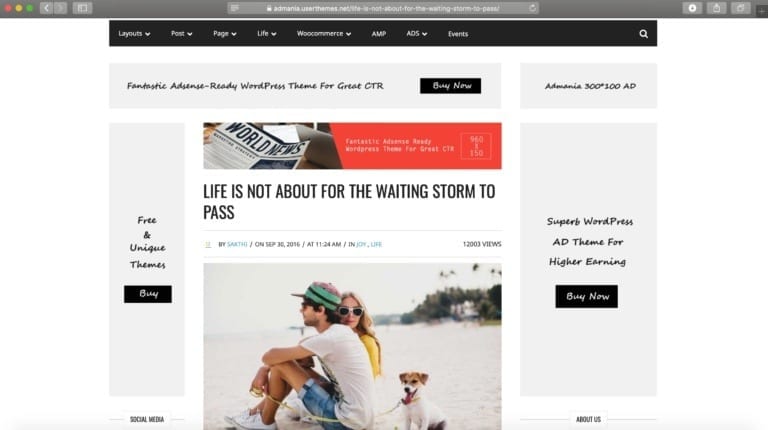Screenshot of a Safari Browser Displaying a WordPress Theme:

The image is a screenshot of a website displayed on the Safari web browser. At the top, the browser has the familiar red, yellow, and green buttons used to close, minimize, and maximize the window. To the left of the address bar, there are grey back and forward navigation buttons, with the forward button being non-selectable. The browser also features a sidebar/bookmark button, an address bar, a download button on the right, and a share button.

The website being viewed is somewhat unclear, but the top of the website shows a black navigation bar with various sections labeled "Layouts," "Post," "Page," "Life," "Commerce," "AMP," and "Ads." There is also a search icon in this navigation bar.

Further down, the content is displayed in light grey boxes with a cursive-like font. One of the messages reads, "Fantastic AdSense Ready WordPress Theme for Great CTR," and there is a button below it that likely says "Buy Now." Another grey box beneath this message reads, "Free and Unique Themes" with another "Buy" button.

The main content area features a large banner ad, including a headline that reads, "Life is not about waiting for the storm to pass." This section also includes a byline, a date, a time, and a view count. The accompanying image shows a couple sitting on a beach; the man is wearing a cap and holding a yellow leash attached to a small dog, while a woman behind him, wearing sunglasses and a yellow shirt, appears relaxed.

To the right, more grey boxes offer additional information. One box seems to say "Academia 300x100 Ad," followed by another box stating, "Superb WordPress Ad Theme for Higher Earning" and another "Buy Now" button. This setup suggests that the website is promoting and selling a WordPress theme designed for high click-through rates and effective advertisement placement.